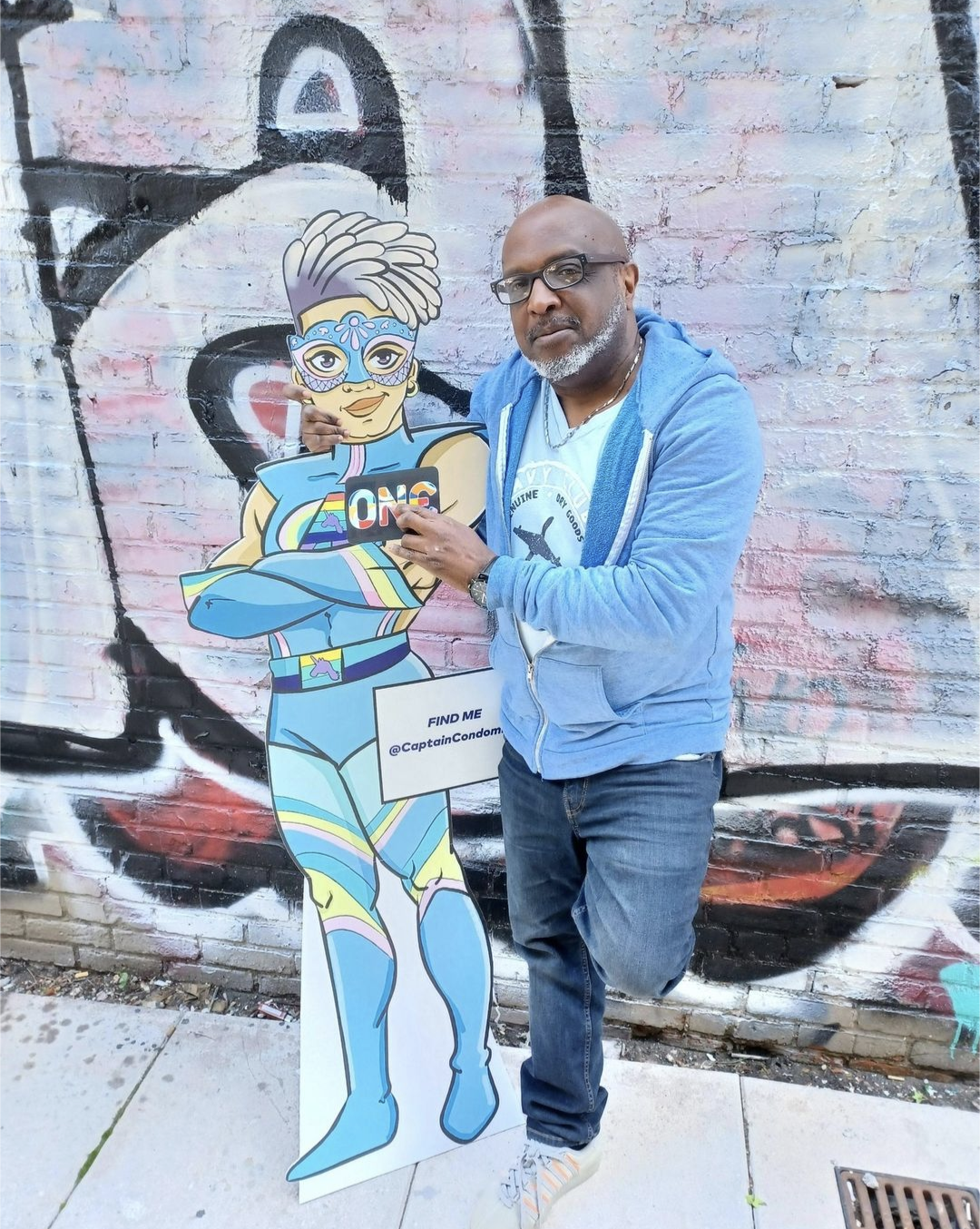This vertical image captures an African-American man standing next to a cardboard cutout of a cartoon superhero. The man is bald with black glasses, a white beard surrounding his chin, and a black mustache. He is dressed in a blue zippered hoodie with white drawstrings, blue jeans, and white tennis shoes. One of his hands is placed on the back of the cutout while the other touches the front. The superhero figure, depicted with short spiky gray hair and a blue mask featuring a silver sequined bottom, wears a light blue sleeveless suit and long gloves adorned with pink, yellow, and blue stripes up to the elbow. The outfit is accessorized with a belt buckle displaying a unicorn. In the background, there is a white and black painted wall covered in graffiti, against which the man is leaning, positioned on a concrete sidewalk with a drain visible in the lower right corner.